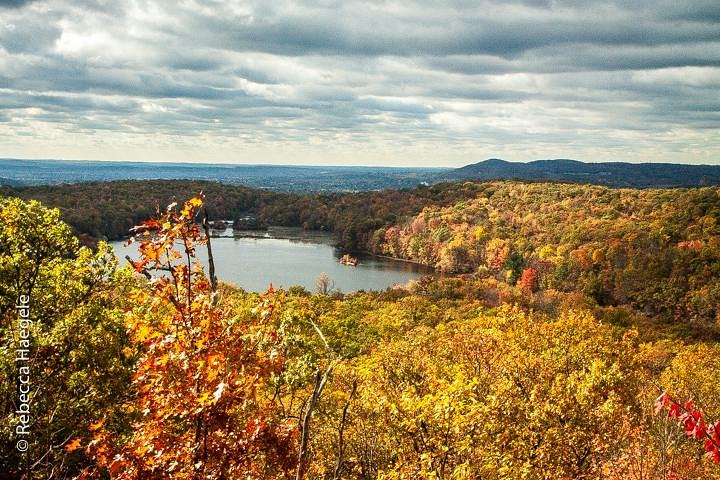This professional aerial photograph by Rebecca Hagele captures a breathtaking autumn scene in a valley dominated by a lake surrounded by a dense forest of trees whose leaves display a vibrant spectrum of red, orange, and ochre hues. The image suggests it was taken in the northeast during the fall season, possibly after or before a rainstorm, as evidenced by the overcast sky filled with low, gray clouds. Despite the cloudy atmosphere, rays of sunshine break through, illuminating the foreground and giving the landscape a dynamic contrast. In the distance, dark mountains rise, their silhouettes softened by the blue haze of atmospheric perspective, enhancing the depth of the scene. The lake, situated toward the back of the photograph, contains what appears to be a small island and possibly a boat on its right side, though it's hard to discern clearly. This expertly composed image, potentially taken from a drone, offers a striking view from above, capturing both the intricate details of the forest canopy and the expansive beauty of the natural landscape.